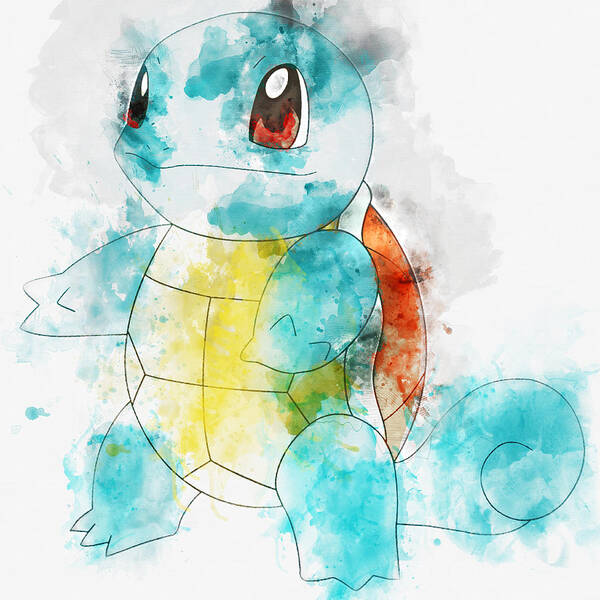The image is a digitally edited artwork of a Pokémon character, specifically a Squirtle, featuring the classic Generation 1 line art style. The character stands on two legs facing to the left and is illustrated with a thin black outline. Instead of solid coloring, the image is marked by a stylized, blotchy watercolor effect, with splotches of blue on Squirtle's head and body, yellow on its stomach, and brown on its shell. The background is a white canvas with some grey around the edges, adding to the painting's dynamic, freeform aesthetic. The coloring appears to be applied haphazardly, giving the impression that it was created with brushstrokes or pastel patted onto the character, creating a lively, textured look without overly strict adherence to the character's outline.